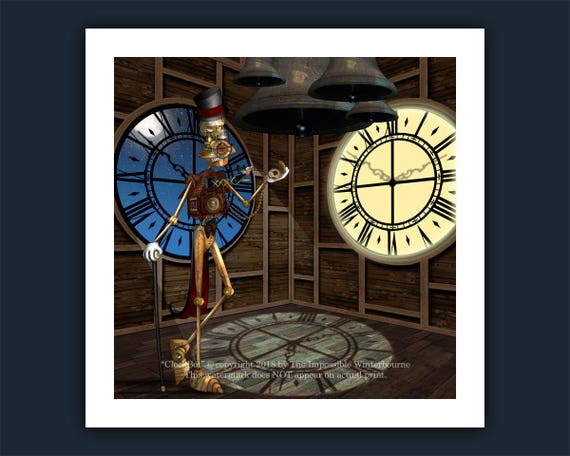The image showcases an intricate, square-shaped painting titled "The Impossible Winter Worn," portraying the interior of a wooden clock tower. At the center stands a mechanical figure known as a clock bot, a humanoid assemblage of brass and various clockwork components. The clock bot features a cuckoo clock for a torso, with a chirping bird emerging from it. Dressed in white gloves and a brown hue, it dons a top hat with a red ribbon and holds a black walking stick in its right hand. The creature's face is composed of clock mechanisms, including a lower jaw and nose fashioned from timepieces, while its left hand clutches an open pocket watch. The wooden walls of the clock tower frame two clocks, one blue and the other white, with their reflections mirrored on the polished wooden floor, illuminated by moonlight filtering through the clock-shaped windows. Overhead, a large black bell is flanked by four smaller ones. The scene is bordered by a thick white frame, with unreadable white text at the bottom against a dark blue background.